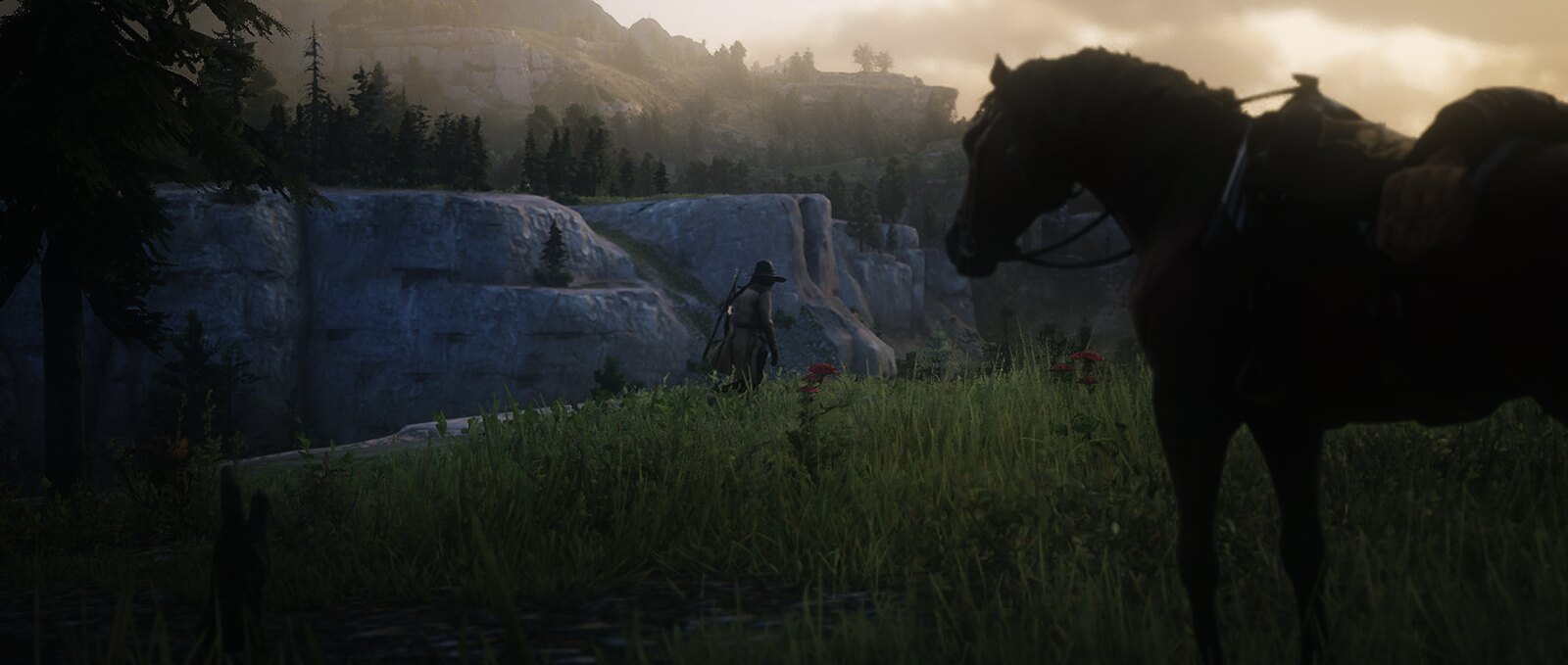In this atmospheric image, a man wearing a hooded green hat is seen walking away from the viewer towards a ridge of gray rocks. To the right of the man stands a dark horse with a saddle on its back. The man is traversing a dark green, weedy grassy area. The scene is shrouded in darkness, but the sky above offers a contrasting light yellowish hue, filled with numerous clouds. At the top of the rocky ridge are numerous trees, and beyond that, a higher hill covered with more trees rises in the background, adding depth to the composition.